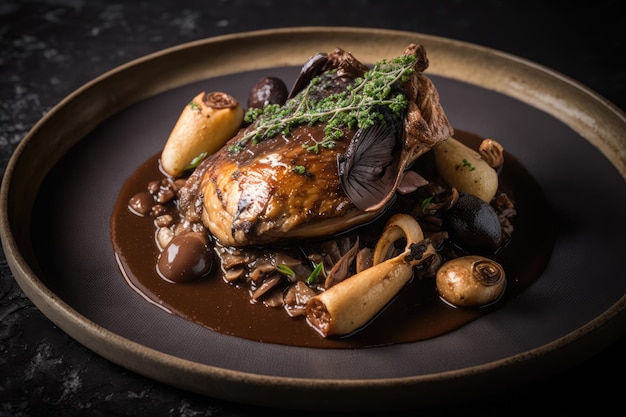A mouth-watering gourmet meal is displayed on a round, brown plate set on a black marble table. The centerpiece of the dish is a succulent cut of meat, possibly chicken or duck, generously drenched in a rich, brown sauce that has a luxurious, chocolatey appearance. Nestled alongside the meat are earthy mushrooms and what appears to be a root vegetable, adding depth to the dish's flavor profile. The monochromatic visual aesthetic, characterized by varying shades of brown and beige, is punctuated by a sprig of fresh green herbs, adding a touch of vibrancy. This casually elegant dinner plate is a delightful fusion of textures and understated colors, promising a delectable gourmet experience.